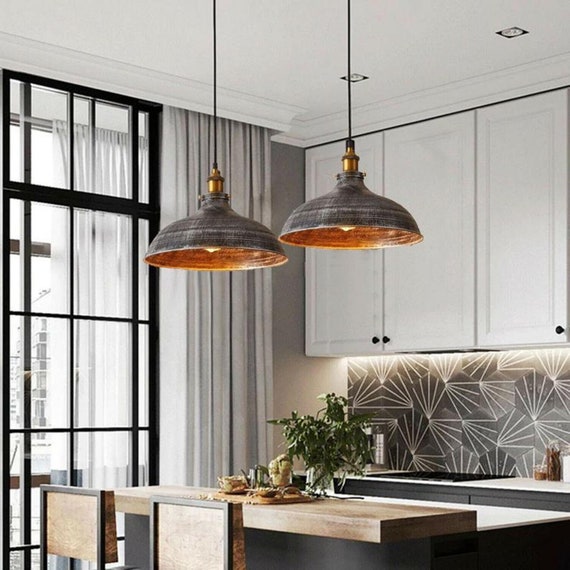This detailed photograph captures a modern kitchen interior, emphasizing the focal point of the design: two distinctive hanging lights. The kitchen features a white ceiling and upper cabinets paired with dark gray lower cabinets. The ceiling also includes round recessed lighting and two large, metal, round lampshades, which hang from black wires over the breakfast bar. These lampshades are dark pewter on the outside, with a bronze interior, adding a unique touch to the otherwise monochromatic space.

The left side of the kitchen showcases a large sliding patio door set in a black frame, adorned with gray curtains that can be drawn from left to right. A cutting board is placed on the central table, accompanied by several chairs neatly tucked in. The wall backsplashes are predominantly white with subtle lines, further enhancing the clean, modern aesthetic. The overall color scheme of the kitchen involves a sophisticated palette of grays, whites, and blacks, with the hanging lights providing a splash of contrasting bronze to create visual interest. The dimmed, disc-shaped lights and the thoughtful combination of colors and textures convey a sleek, contemporary style suitable for showcasing on a high-end interior design website or a lighting retail platform.